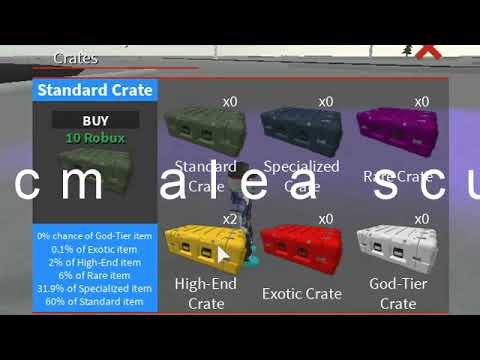The image appears to be a screenshot from a video game screen that displays options for purchasing loot crates. In the upper left hand corner, the screen reads "Crates" with a red line below it, followed by the text "Standard Crate - Buy 10 Robux." Centrally, there is white text extending across the screen spelling out "C-M-A-L-E-A-S-C-U." In the lower left corner, a small blue box lists the item probabilities: 0% chance for a god tier item, 0.1% chance for an exotic item, 2% chance for a high-end item, 6% chance for a rare item, 31.9% chance for a specialized item, and 60% chance for a standard item. To the right of this box, there are six colored crates arranged in two rows. From left to right, the top row includes a green crate (standard), a black crate (specialized), and a purple crate (rare). The bottom row features a yellow crate (high end), a red crate (exotic), and a white crate (god tier). Some crates have text indicating quantities, such as "x2" on the yellow one.